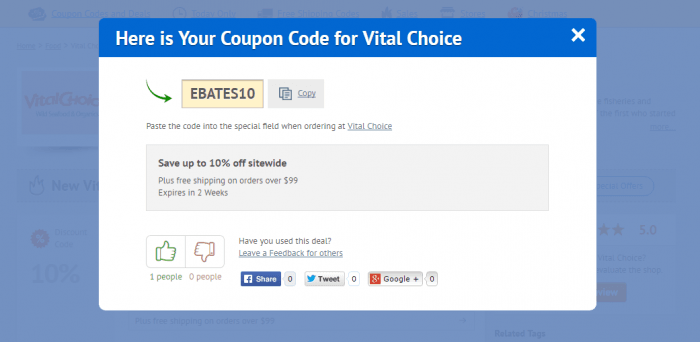The image showcases a promotional pop-up box that appears on a computer screen. The pop-up features a blue header with an 'X' button for closing. The main section announces a coupon code for Vital Choice against a beige background, prominently displaying "Ebates10." Next to the code is a "Copy" button for easy duplication. The instructions advise users to paste the code into the specified field when ordering on the Vital Choice website.

Additional details include a gray box outlining the offer: save up to 10% off site-wide, plus free shipping on orders over $99, with an expiration date in two weeks. The pop-up also features user engagement options, showing that one person rated it as helpful with a thumbs-up, while no one rated it negatively. There's a prompt asking, "Have you used this deal? Leave feedback for others," indicating that only one person has used the deal so far.

Social sharing options are available, allowing users to share via Twitter or Google, though each currently displays zero shares. Faded in the background, the blue-shaded Vital Choice website is visible, with its orange logo partially seen on the left side of the pop-up box, indicating the pop-up appeared when accessing the site. This promotional pop-up highlights the brand's effort to offer additional savings and engage with customers.